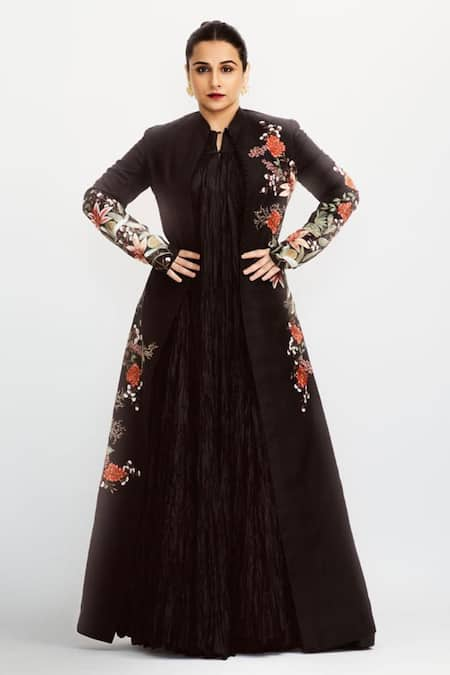The image depicts a model standing against a white background, posing with both hands confidently placed on her hips. She gazes directly at the camera. The model has a light tan complexion, prominent arched eyebrows, dark eye makeup, and striking red lipstick. Her dark hair is parted in the center and styled into a low bun. She also adorns gold earrings.

The model is showcasing a floor-length black overcoat featuring intricate floral appliques in red, white, and green on the left breast, the lower sleeves, and the sides of the coat by the legs. Beneath this garment, she wears a crinkly-textured black dress that adds to the outfit's elegance. The overall brightness and clarity of the image highlight the details of the model and her attire.